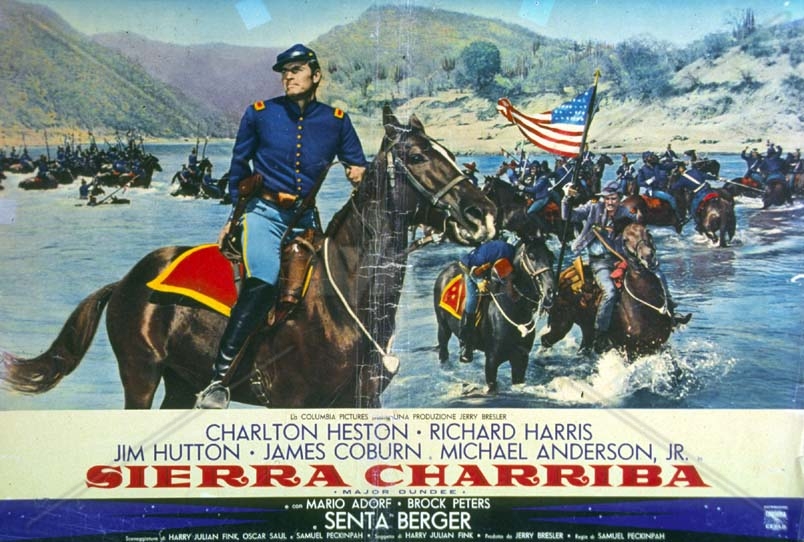This image is an advertisement poster for a historical movie set during the American Civil War. Featured prominently in the center, a military troop in blue uniforms with black boots and yellow buttons is seen crossing a rippled, blue waterway on horseback, while carrying an American flag. In the distance, green grassy land, multiple mountain ranges, and a clear blue sky create a picturesque backdrop. The bottom of the poster lists the starring actors: Charlton Heston, Richard Harris, Jim Hutton, James Coburn, and Michael Anderson Jr. in blue text. Below that, the names Mario Adorf, Brock Peters, and Cinta Berger appear in white text on a blue and black background. The poster is identified as a production by Columbia Pictures, with the film title "Sierra Charriba" mentioned in red text.